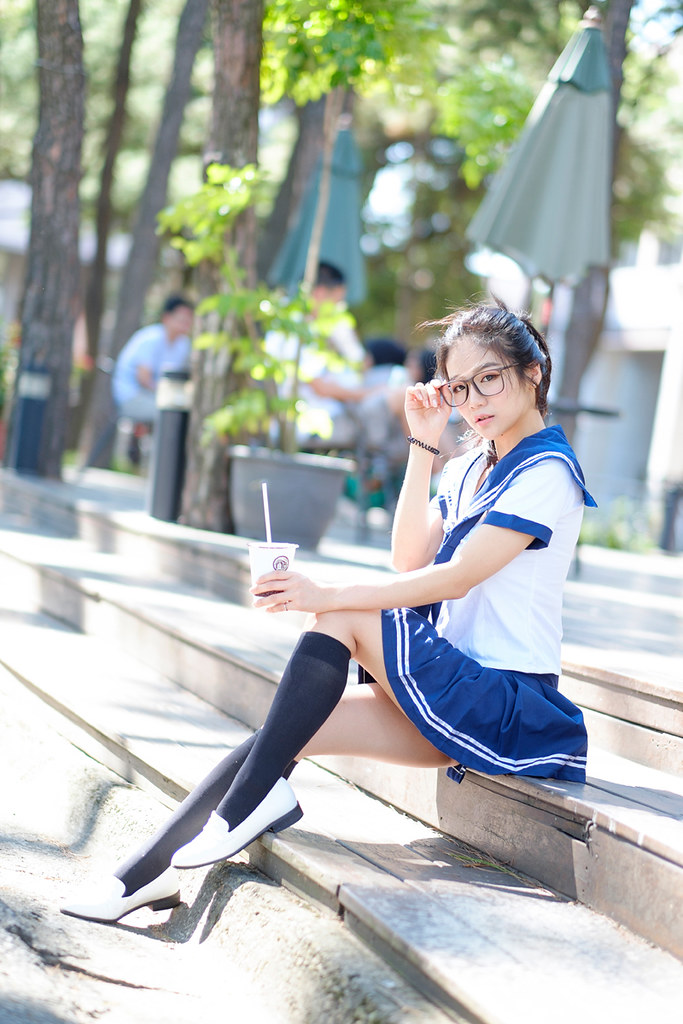A young woman, possibly 16 or 17 years old, is sitting on stone steps outside on a bright, sunny day. She has a light skin complexion and black hair pulled back, possibly into a ponytail, and she wears large, dark-framed glasses. She is dressed in a sailor-style school uniform featuring a white shirt with blue trim around the sleeves and collar, paired with a dark blue skirt that has circular white stripes and reaches mid-thigh. She has short black stockings pulled up just below her knees and white, low-heeled loafer-type shoes. Her right arm is raised, adjusting her glasses, and she wears a black bracelet on her right wrist. With her left hand, she holds a cup that appears to have a Starbucks logo on it. The scene includes background details such as blue umbrellas, potted leafy plants, and other people sitting at tables, though they are blurred to keep the focus on her. The setting is characterized by ample natural sunlight, enhancing the clarity and brightness of the image.